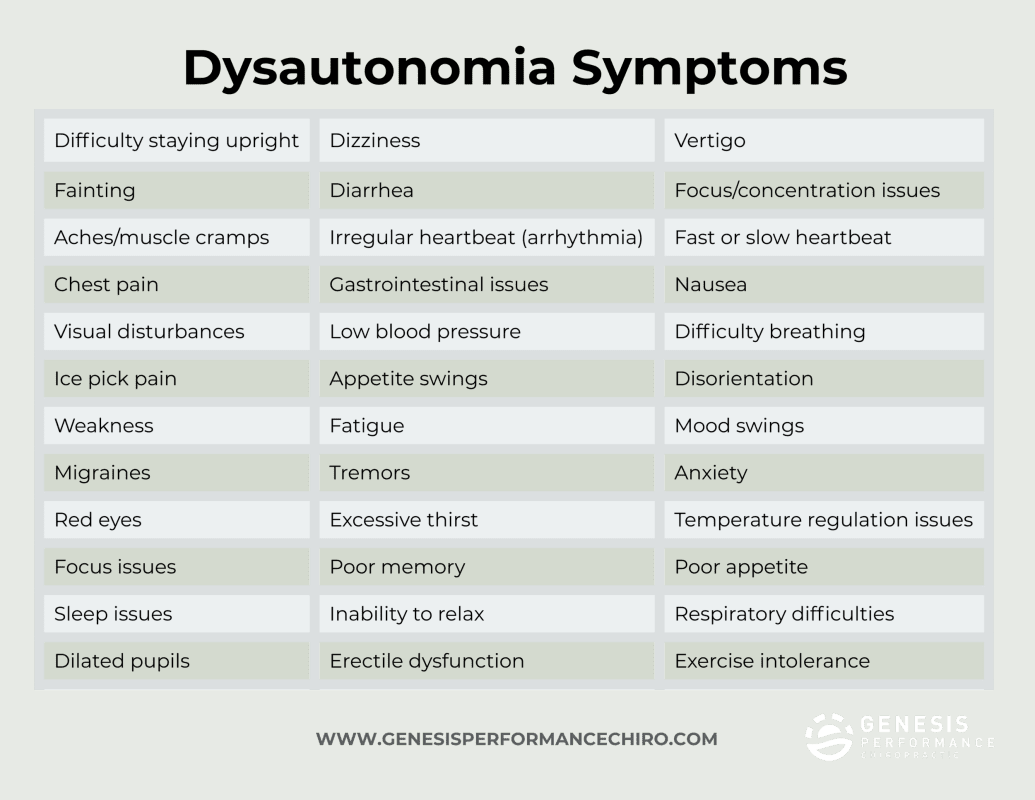**Detailed Caption for Dysautonomia Symptoms Chart:**

The image features a square background with a taupe color that has a subtle green tinge. At the top center, in bold, it reads "Dysautonomia Symptoms," with "Dysautonomia" and "Symptoms" starting with capital letters. Below this title, a chart is presented, alternating between darker gray and two shades of taupe with a greenish undertone as background colors for different sections.

This organized chart lists the symptoms associated with dysautonomia, categorized as follows:

1. **Difficulty staying up at night**
2. **Fainting**
3. **Aches and muscle cramps**
4. **Chest pain**
5. **Visual disturbances**
6. **Ice pick pain**
7. **Weakness**
8. **Migraines**
9. **Red eyes**
10. **Focus issues**
11. **Sleep issues**
12. **Dilated pupils**
13. **Dizziness**
14. **Diarrhea**
15. **Irregular heartbeat**
16. **Gastrointestinal issues**
17. **Low blood pressure**
18. **Appetite swings**
19. **Fatigue**
20. **Tremors**
21. **Excessive thirst**
22. **Poor memory**
23. **Inability to relax**
24. **Erectile dysfunction**
25. **Vertigo**
26. **Locus in concentration issues** (emphasized)
27. **Faster or slow heartbeat**
28. **Nausea**
29. **Difficulty breathing**
30. **Disorientation**
31. **Mood swings**
32. **Anxiety**
33. **Temperature regulation issues**
34. **Poor appetite**
35. **Respiratory difficulties**
36. **Exercise intolerance**

At the bottom of the image, the URL "www.genesisperformancechiro.com" is provided for further information.